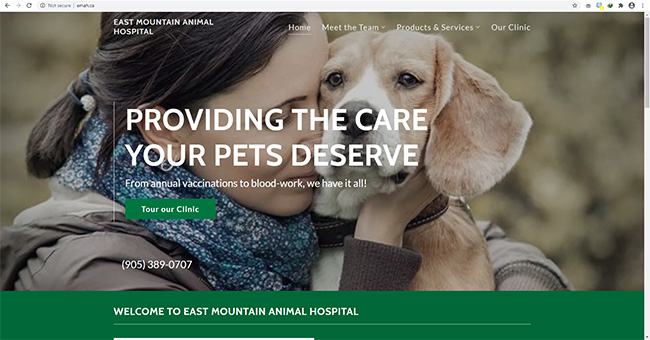The screenshot depicts the homepage of the East Mountain Animal Hospital website, captured through a whole-screen snapshot that includes the entire browser interface. Although the URL isn't clearly visible due to the zoom level, essential details of the page are discernible. Dominating the homepage is a touching photograph of a woman, with short brown hair in a ponytail, warmly embracing a beagle. The setting appears to be in the fall or winter, as indicated by the woman's attire—a jacket and a light scarf. The beagle, adorned with a collar, gazes into the distance while the woman's eyes are closed, sharing a serene moment of connection.

Bold white text overlays the image, promoting the clinic's range of services: "Providing the care your pet deserves from animal vaccinations to blood work. We have it all." Just beneath this message is a prominent button labeled "To Our Clinic," likely a call-to-action for visitors. The clinic's contact information is clearly listed: 905-389-0707.

Further down the page, a welcoming message reads, "Welcome to East Mountain Animal Hospital." The primary navigation menu is also partially visible, featuring options such as "Meet the Team," "Products and Services," and another button titled "Our Clinic." Overall, the screenshot captures a warm and inviting introduction to the veterinary services offered by East Mountain Animal Hospital.